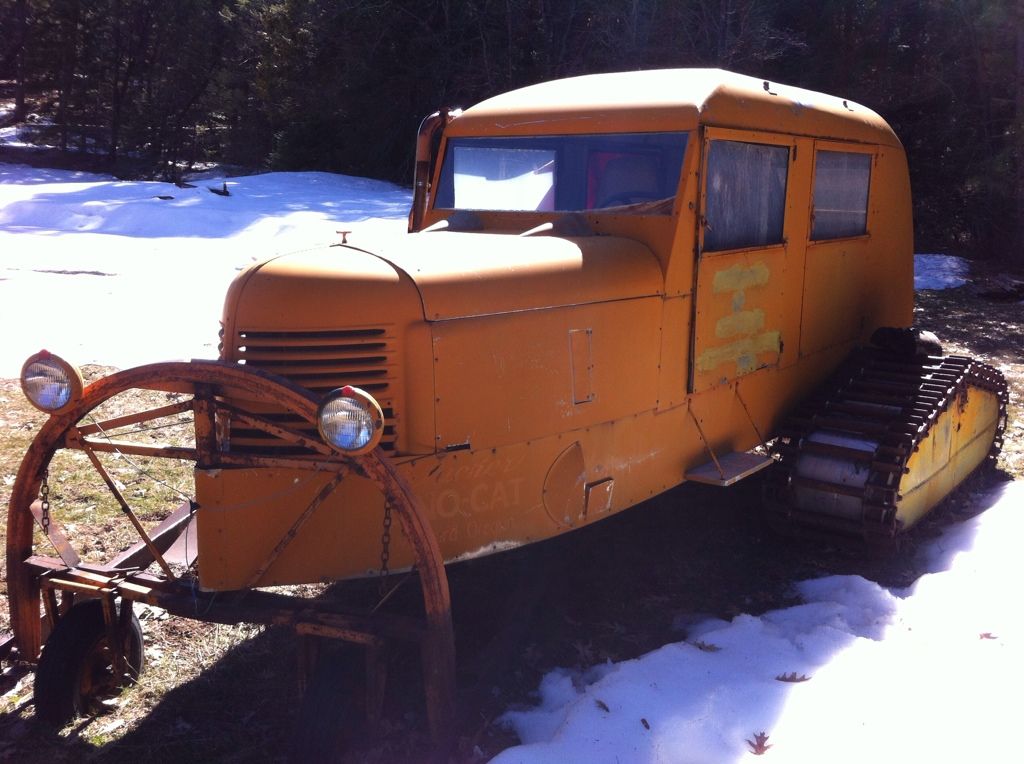This image features an advertisement for the website Photobucket, prominently centered with the text "Photobucket: Protect more of your memories for less." The focal point of the image is an old vehicle that resembles a hybrid between a car and a tractor, characterized by its brown-orange color and bulldozer tracks instead of traditional tires. The vehicle, equipped with two small headlights and windows, occupies the middle portion of the photo. The background sets a rustic scene with snow-covered ground reflecting sunlight and a backdrop of woods with visible tree trunks and shrubs, suggesting the vehicle is situated in a farm-like or wooded area. This ad emphasizes the ease and security of preserving your precious memories, like a photo of this vintage vehicle, using Photobucket.